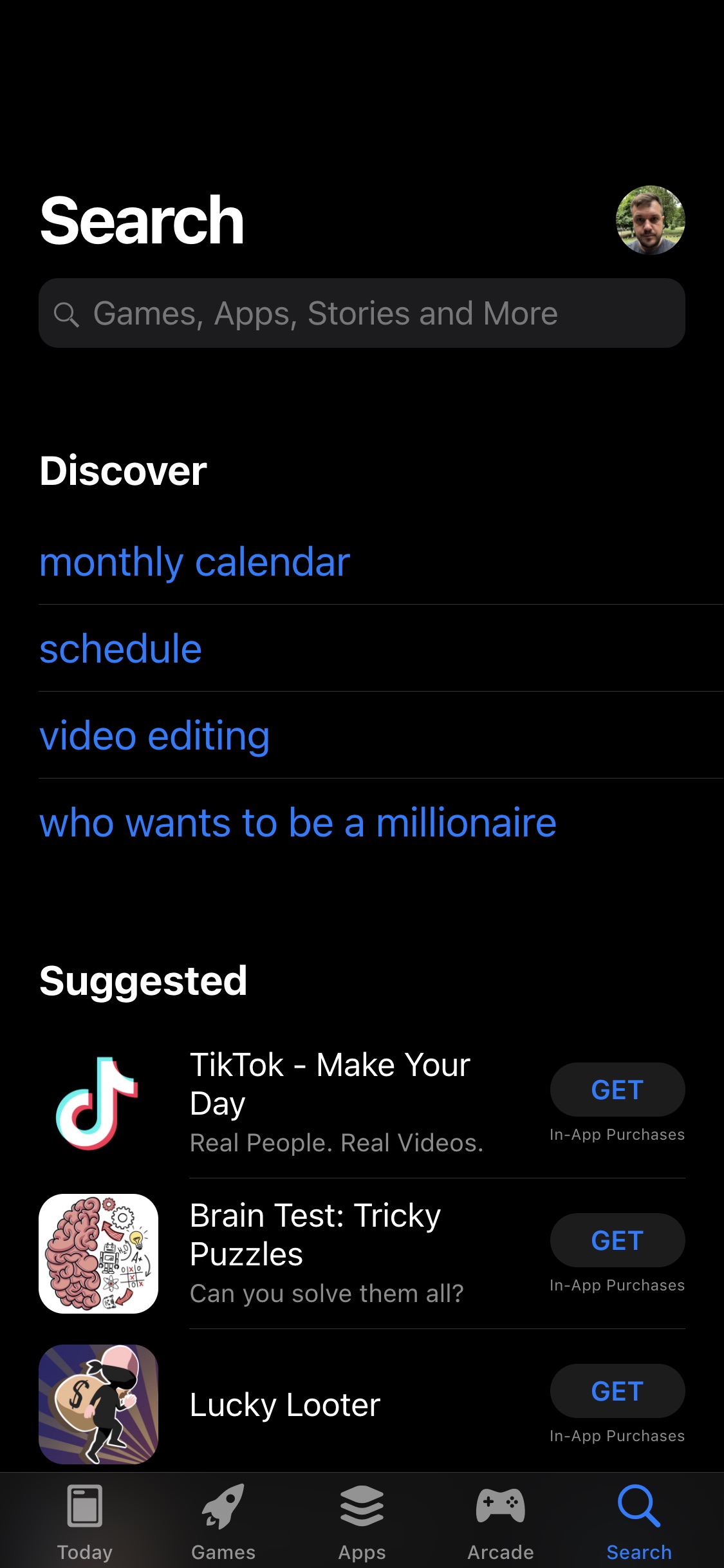The image features a black background with white text. At the top left corner, there is the word "Search". On the right side, there is an image of a man, and below that, a gray circle containing a magnifying glass icon. Below this, the text "Games, Apps, Stories, and More" appears in white font.

Further down, the text "Discover" is displayed in white, followed by blue text listing several items: "Monthly Calendar", "Schedule", "Video Editing", and "Who Wants to Be a Millionaire". Below these items, "Adjusted" is written in white font.

On the left side of the image, there is a TikTok logo in white. Next to it, the text "TikTok - Make Your Day" appears, with the tagline "Real People. Real Videos." written in lighter font underneath. Below this, a blue "Get" button is accompanied by the note "In-App Purchases" in gray.

Following this, there is an icon of a white square that might be pink, accompanied by the text "Brain Test: Tricky Puzzles – Can You Solve Them All?" in white. Again, a blue "Get" button with "In-App Purchases" is displayed.

Further down, an illustration of a person in black holding a yellow money bag with a pink hat on a purple background appears. To the right of this image, the text "Lucky the Looter" is shown, along with another blue "Get" button and "In-App Purchases".

At the bottom of the image, several icons with corresponding labels are displayed: "Today" with a calendar icon, "Games" with a rocket ship icon, "Apps" with three long squares stacked on top of each other, "Arcade" with a game controller icon, and "Search" in blue text with a blue magnifying glass icon above it.